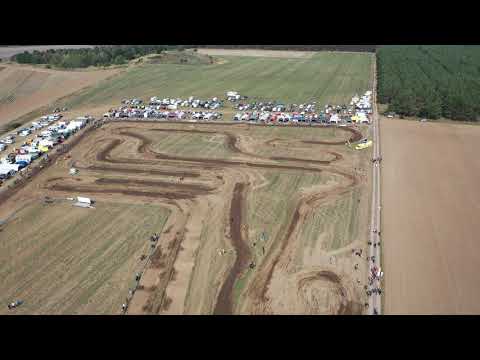An aerial drone photograph captures a rectangular parcel of farmland repurposed as a dirt race track. This high-angle shot showcases a complex network of winding dirt trails, including sharp bends and hairpin turns. The track's brown, soil-covered paths interweave through green fields, creating striking contrast. Surrounding the dirt track, numerous RVs, trucks, and cars are parked along the perimeter, particularly concentrated on the right-hand side where a dirt road runs parallel. A gathering of spectators is visible near this road, albeit indistinct due to the image's poor resolution. The broader landscape features additional fields, some verdant and others barren, with patches of pine trees dotting the distance.